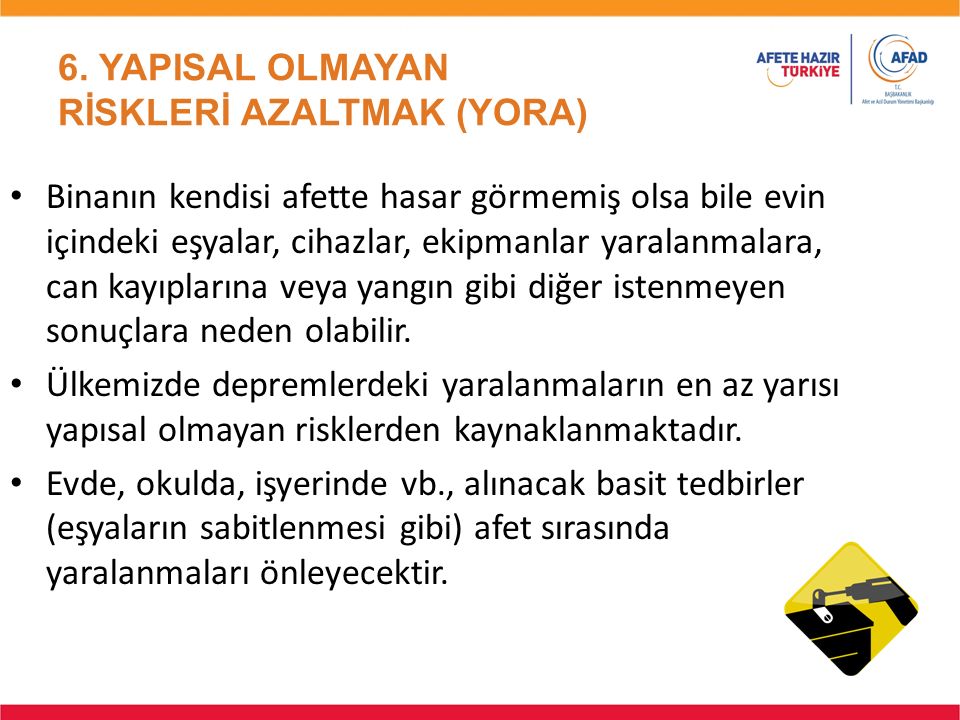The image portrays an informative slide, distinguished by an orange banner at the top and a red banner at the bottom. Dominating the top portion, orange text spells out "SIX" in all capital letters, followed by three bullet points of black text in a sans serif font. The entire text is in a non-English language and includes phrases like "EFEDI, HAZAR, TURKEY, AFAD."

The focal point in the bottom right corner is a detailed illustration of a gray and black screwdriver attaching a bracket to the top of a black dresser. This piece of furniture is being securely mounted to a yellow wall. The brackets are shown fastening the dresser to the wall, emphasizing safety and stability. The entire scene appears to be an instructional guide on securing furniture to prevent accidents.